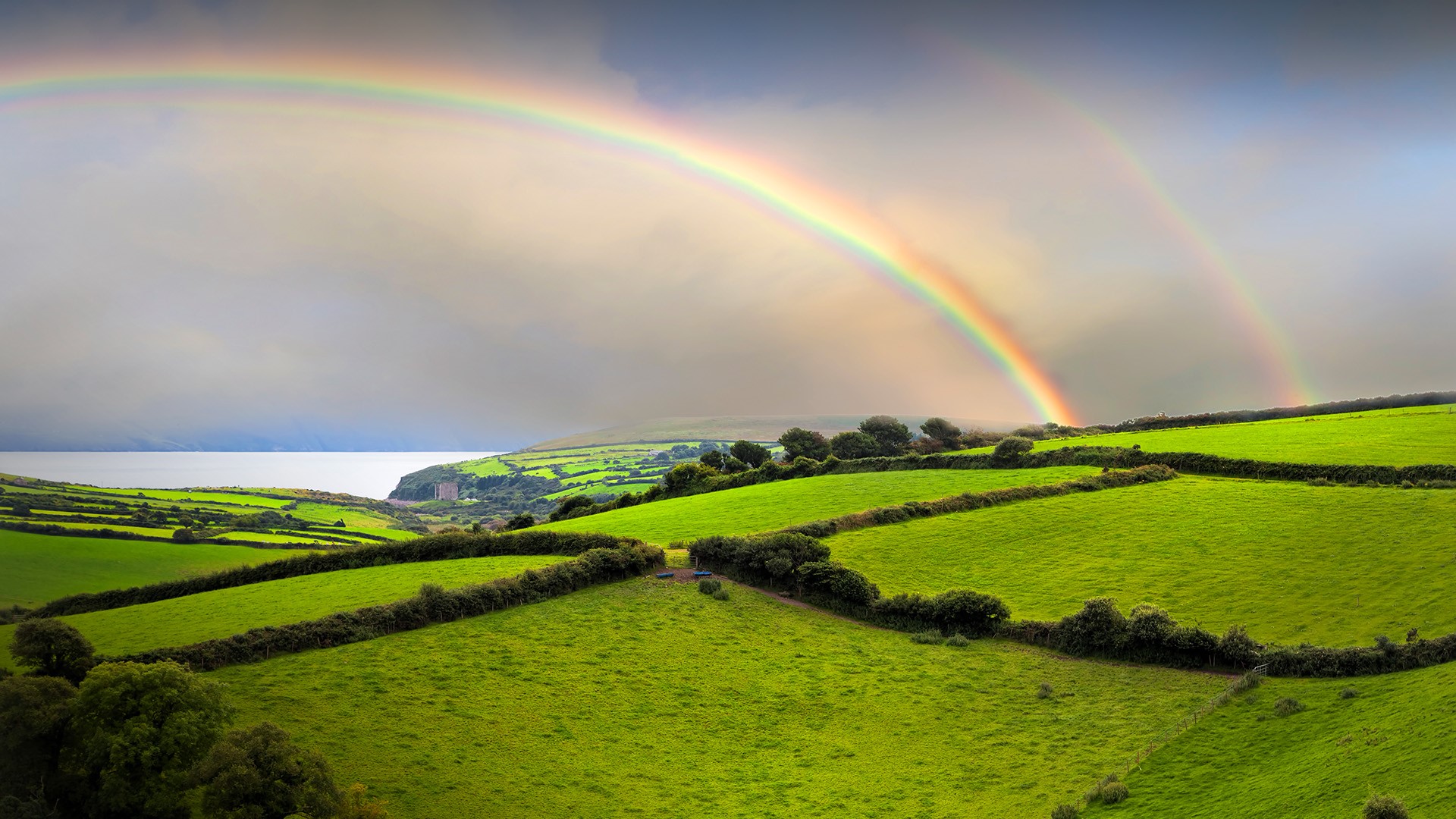This image depicts a picturesque aerial view of a rolling countryside, reminiscent of Ireland's grassy shires. The vibrant, light green fields are divided by small, darker tree lines creating a patchwork of parcels. Among these parcels, roughly five distinct squares of trees stand out, with more scattered towards the left. The scene is framed by overcast skies, predominantly cloudy with patches of blue peeking through, marking a typical mix of weather. In this dramatic sky, a double rainbow arcs across the landscape; the lower, more vivid rainbow shows the full ROYGBIV spectrum, while the higher, fainter rainbow lies just to its right. The rainbows seem to merge into the fertile land without visible endpoints. In the distance, where the rolling hills descend, we see a cliff edge overlooking a large, subtly lit body of water, appearing white due to the lighting. This scenic view beautifully captures the tranquil and lush nature of the countryside.